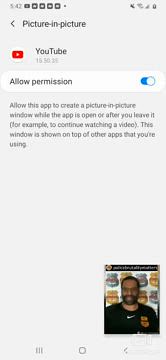Here's a cleaned-up and detailed descriptive caption for the image:

"A photo of a smartphone screen displaying an app permission setting. At the top left of the screen, the current time and several notification icons are visible. In the top right, additional icons likely include signal strength, Bluetooth status, and the battery percentage. Below these icons, a back arrow and the text 'Picture-in-Picture' are shown, followed by the red YouTube logo and the text 'YouTube' next to it. Underneath, there is a toggle button set to the 'on' position, allowing permission for the YouTube app to create a picture-in-picture window. The text explains that this enables the app to continue showing a video overlay even when the user is multitasking. 

Towards the bottom right of the screen, there's a small video thumbnail showing what appears to be an African American man with facial hair, wearing a black shirt with a white Nike swoosh and a matching logo on the chest. Although the background of the video is unclear, it might contain team logos. At the very bottom, the screen displays navigation buttons including a home button, a possible pause button, and a back button."